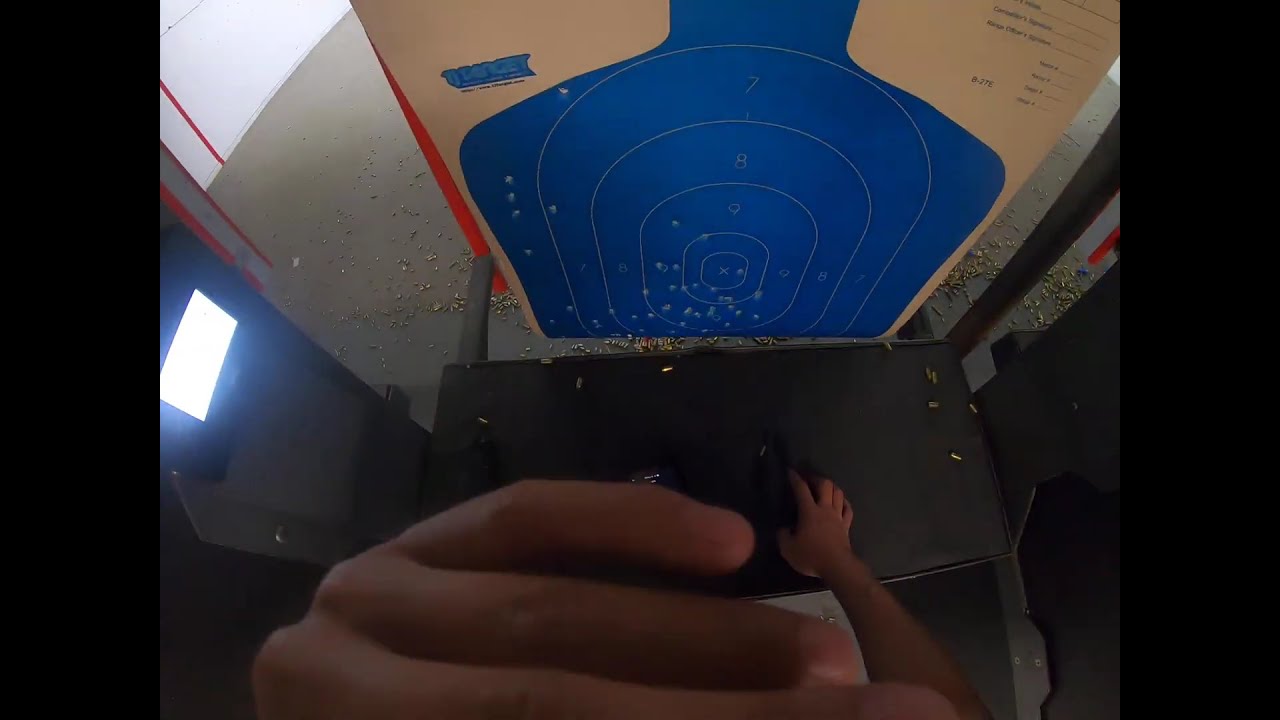The photo captures a horizontal scene at a shooting range, framed by thick vertical black borders on each side. Dominating the foreground is a person's left hand, raised near their face, while their right hand grips a pistol resting on a black shelf. The background reveals a blue paper target with a human body outline, attached to a brown cardboard backing. This target features numerous bullet holes, concentrated largely around the edges and lower sections. Surrounding the target on the concrete floor are countless bullet casings, adding to the stark atmosphere. To the left, a bright square light source illuminates part of the scene, while the target itself appears numbered, indicative of a detailed shooting practice evaluation.